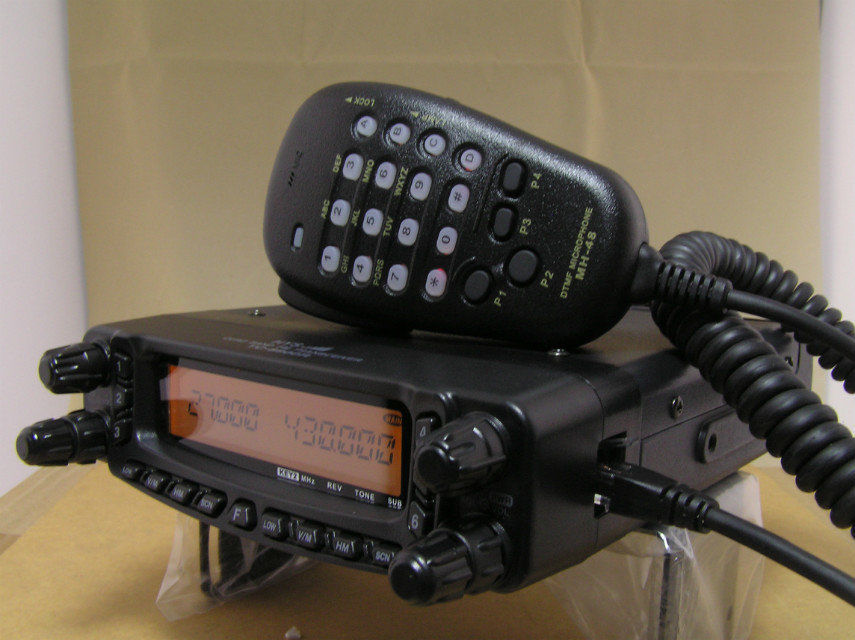This indoor photograph features a sophisticated black radio device, likely resembling a CB radio or a specialized communication system. The main console, which rests atop a wooden structure, is equipped with an orange digital screen displaying the numbers "27000" followed by "430000." The device includes four knobs and a row of white buttons. Additionally, there are black buttons labeled P1, P2, P3, and P4. A controller panel, which rests on top of the main unit, features a myriad of white buttons numbered from 1 to 9, followed by 0, and includes special symbols such as an asterisk (*) and a pound sign (#). It also has buttons labeled A, B, C, and D. Several black cords are connected to the device, including one that appears to be an Ethernet cable. There are visible labels near the screen with unclear text, possibly saying "REV," "TONE," and "SUV." In the background, a cardboard box and an unidentified paper on the wall can be seen. The entire setup is partially wrapped in plastic, indicating either newness or a temporary setting.